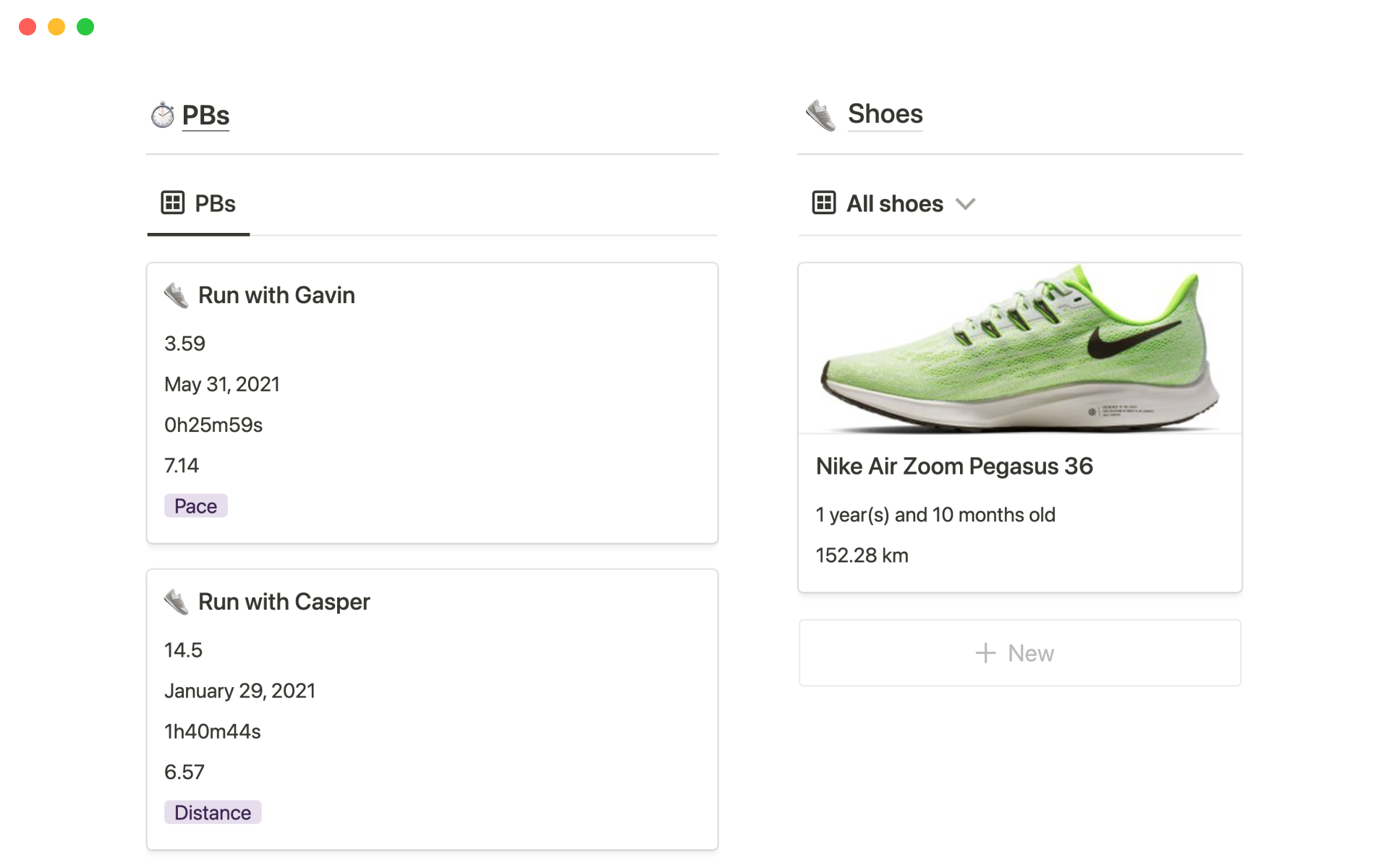A website screenshot features an inventory and tracking interface for running shoes. The image is horizontally oriented and portrayed against a seamless, white background consistent with the screen's backdrop, devoid of any borders. In the upper left corner, three filled circles (red, yellow, and green) are visible, simulating window control buttons, typical of a web browser interface. Below this area, an icon of a clock can be seen, next to bold black text reading "PB's," underlined by a thin black line.

Adjacent to "PB's" on the right side, an icon of a shoe is displayed, with the text "Shoes" beneath it, similarly underlined. Separating each section are an arrangement of lines, providing clear demarcation. 

Further down, a smaller square icon next to "PB's" is followed by another icon featuring a box with a shoe inside, paired with the text: "Run with Gavin, 3:59, May 31, 2021, 0 hours 25 minutes 59 seconds, 7:14," with the term "Pace" highlighted in a purplish background. Below it, similar details for "Run with Casper, 14.5, January 29, 2021, 1 hour 40 minutes 44 seconds, 6:57," with the word "Distance" selectively highlighted in purple.

Lower down, under the section labeled for "All Shoes," appears the image of a green Nike Air Zoom Pegasus 36 shoe. The description lists its age as "1 year, 10 months," with a total distance of "152.28 kilometers" covered, accompanied by a clickable plus sign that suggests the option to add a new shoe.